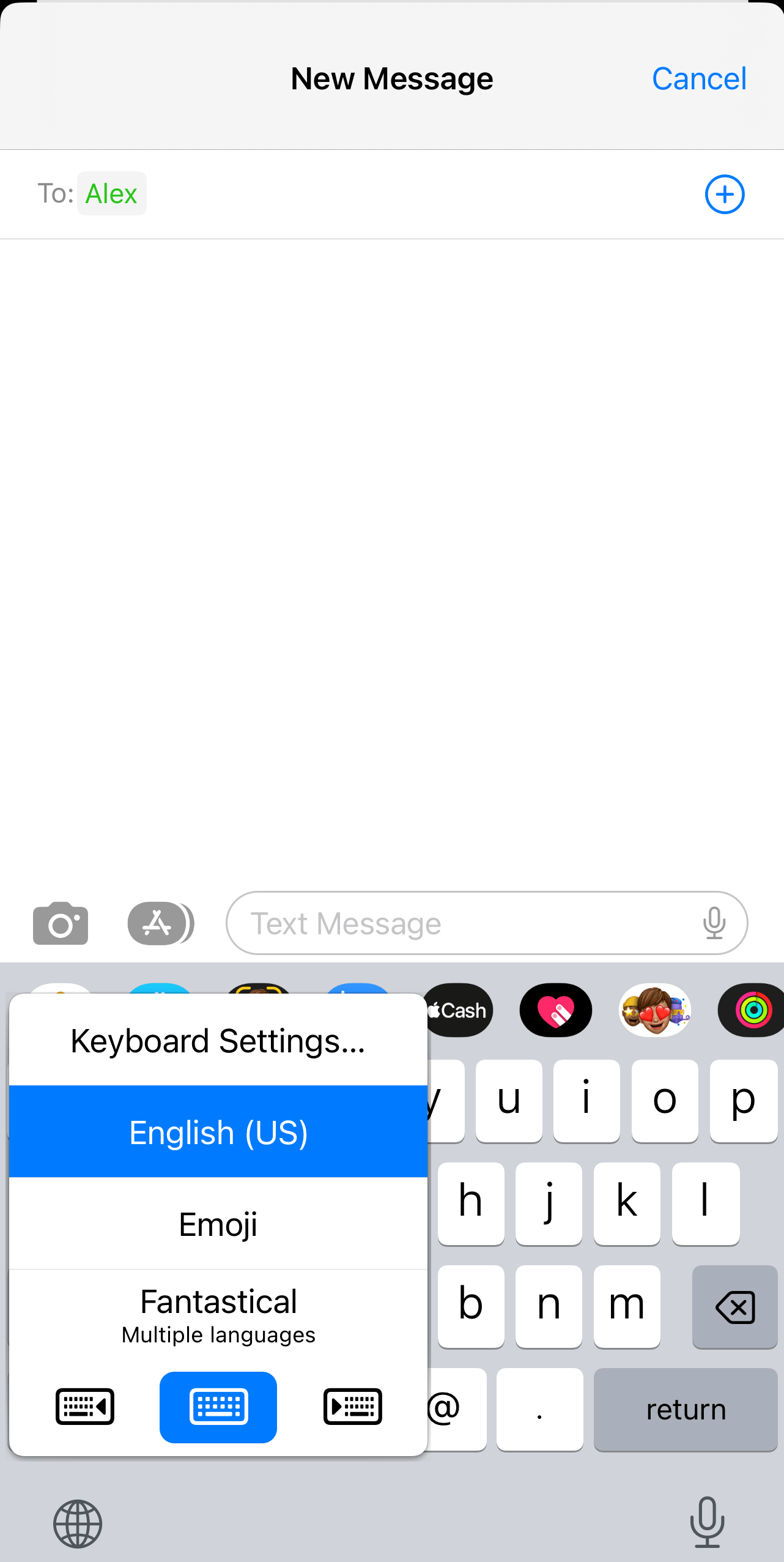This image displays a screenshot of a messaging app interface against a white background. At the top of the screen, a small blue box with the text "New Message" in black is visible, accompanied by a blue "Cancel" option. Both top corners of the image feature small black areas. Below this section, the recipient field labeled "To: Alex," highlighted in green, is presented next to a blue plus sign enclosed in a circle.

Beneath this, a predominantly white screen appears, including a camera icon and a small gray circle containing the letter "A." The text message input block is situated here as well. A dropdown menu in a white box is also included, displaying options such as "Keyboard Settings" and "English (U.S.)" in a blue box. 

Additional options listed are emojis, the "Fantastical" keyboard, and other multi-language keyboards. Among the three visible keyboard selections, the middle one is highlighted in blue. The regular keyboard interface is displayed on a light blue background with several icons at the top. At the bottom, the return key is shown, with a blue section below it containing a globe icon in the left corner and a microphone icon in the right corner.